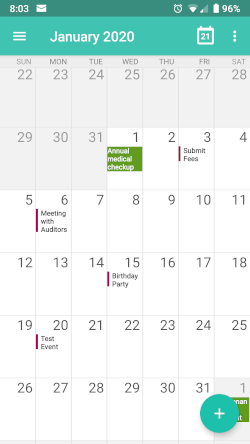The image features a white background with various colored boxes and text. At the top, there is a dark green box displaying the number "803," an envelope icon, and a battery status showing 96%. Below it, a lighter green box has three horizontal lines, an inscription that reads "January 2020," and a small white box with a green interior and the number "21" in white text, accompanied by three white dots.

The calendar layout follows, with light blue boxes representing the dates from the 22nd to the 31st. The 1st is shown against the white background. Specific dates are highlighted with colored lines indicating events:

- The 1st has a green box labeled "annual medical checkup."
- The 3rd features a red line with the text "submit feeds."
- The 6th shows a red line titled "meeting with auditors."
- The 15th includes a red line denoting a "birthday party."
- The 20th has a red line labeled "test event."

At the bottom, between the 31st and the 1st of the next month, there's a notable green circle with a white plus sign, which signifies the creation of a new event. The 1st of the following month is marked by a green box.